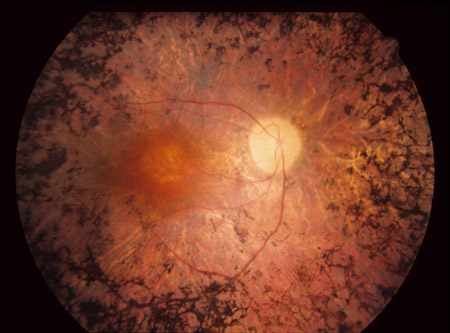The image depicts a circular, colored photograph set against a black background. It features what appears to be a translucent, organic structure, resembling either an underwater jellyfish, an internal structure of a human eye, or an embryonic form. The background is mostly light orangish-pink, and the object itself contains intricate, vein-like lines running throughout.

At the center-left, there is a faint orange splotch, suggesting a highlighted area or an internal feature. This part is described as either a jellyfish's spine, an eye's veins, or another internal detail. Adjacent to this is a misshapen, lighter circle, almost white to cream-colored, adding to the complexity of the central features.

The image also has blackish dots along the edges that fade towards the center, enhancing the sense of depth. The subtle, network-like lines that flow from the edges inward add to the impression of veins or spines, contributing to its intricate appearance. The photograph captures the organic intricacies with a glowing central area, providing a detailed, almost ethereal visual.